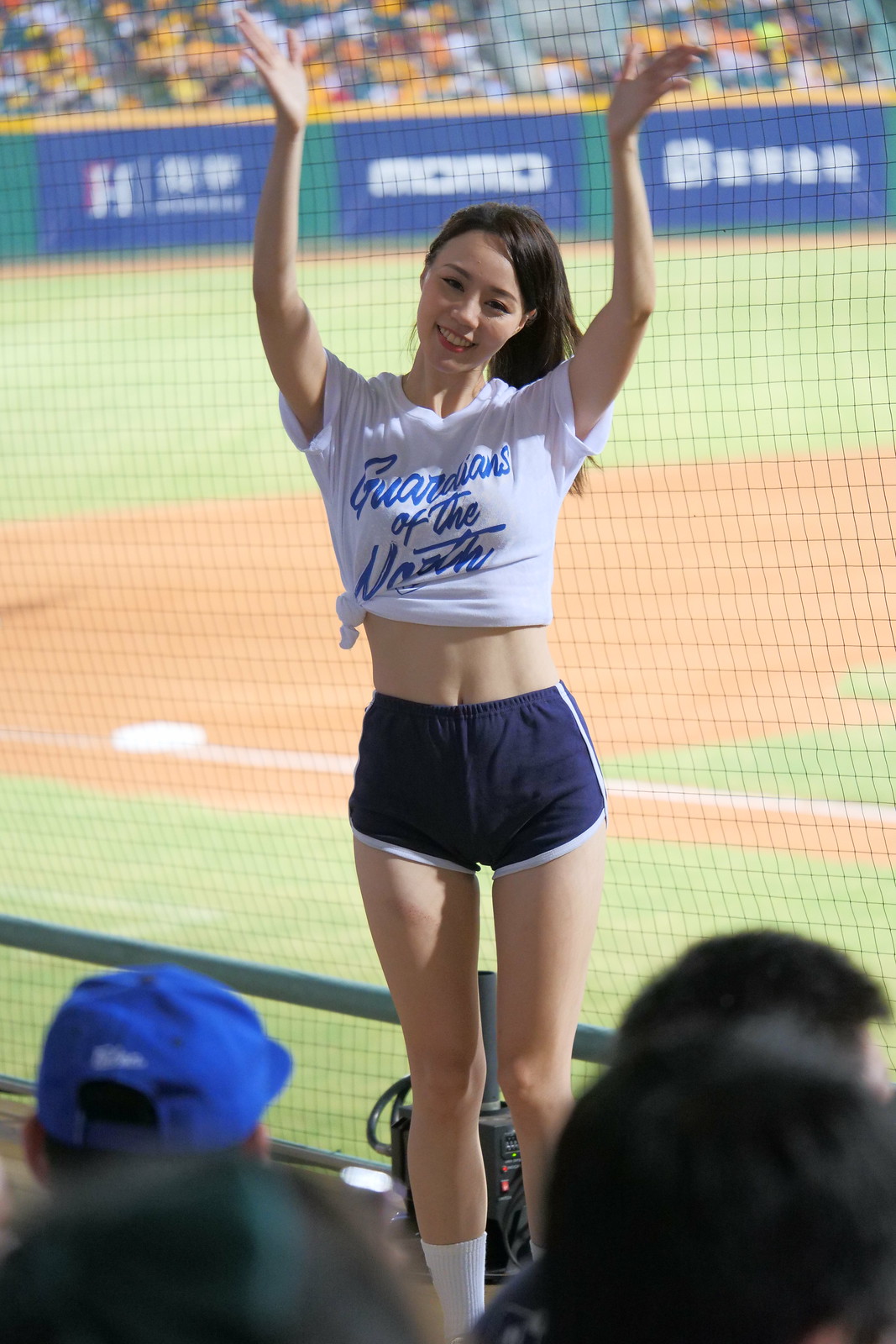The image is a color portrait photograph capturing a lively scene at a baseball game. The central focus is a cheerful young cheerleader, likely a Japanese teen, standing in front of a blurred baseball field. She has long, dark hair, and her arms are raised above her head, clapping with a bright smile on her face. She is facing the camera directly, though her head tilts slightly to the left. The cheerleader is dressed in dark blue, form-fitting shorts with white trim and a white t-shirt tied off to expose her midriff. The shirt features blue text that reads "Guardians of the North." 

In the foreground, the backs of several spectators seated in the bleachers are visible, all blurred to keep the cheerleader as the focal point. One of the spectators is wearing a blue baseball cap. The background details include a light green grass field, brown dirt, white base, and baseline, with a blue and green fence adorned with white advertisement text. This cohesive scene combines the elements of a bustling sports environment with the energetic presence of the cheerleader, all portrayed with photographic realism.